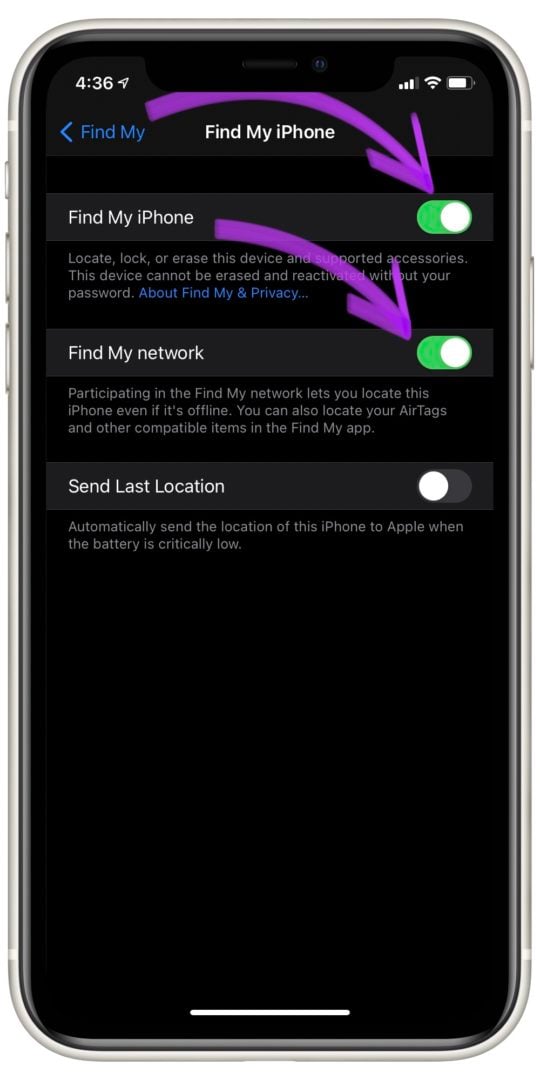In this vertically rectangular image of a cell phone, the device is shown in portrait orientation with its rounded corners visible. The screen primarily displays a black background. The top-left corner indicates the time as 4:36 in white text, while the upper right corner shows icons for the signal bar, Wi-Fi, and battery status, aligned from left to right. Centered on the screen is the title "Find My iPhone," suggesting that this is a setting or instructional display.

Directly below the title, the image features a drop-down list with three options: "Find My iPhone" and "Find My Network," both of which have their toggles switched to the on position, and "Last Location," which has its toggle switched off. Two prominent purple arrows, originating from the left side of the image, point directly to the toggles for "Find My iPhone" and "Find My Network," emphasizing their active status. The overall presentation suggests that this is an instructional or tutorial image, guiding the viewer on how to enable specific settings within the "Find My iPhone" feature.